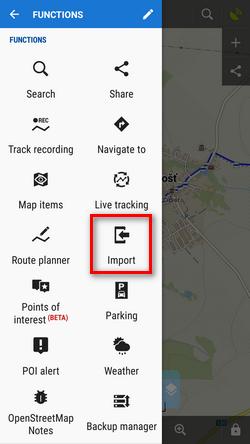The image features a comprehensive menu interface with a blue border adorning the top. At the top left, there is an arrow icon pointing to the left followed by a white, all-uppercase text that reads "FUNCTION." Adjacent to this text on the right, a pencil icon is displayed, and below it, "FUNCTION" is repeated in smaller blue uppercase letters.

Beneath this section, a series of options are listed with corresponding icons:

1. "SEARCH" accompanied by a magnifying glass icon.
2. "SHARE" depicted with three interconnecting circles and two connecting lines.
3. "TRACK RECORDING."
4. "NAVIGATE TO" next to a black diamond with a right-pointing arrow.
5. "MAP ITEMS" positioned to the left, while "LIVE TRACKING" is on the right.
6. "ROUTE PLANNER" on the left, with "IMPORT" on the right, illustrated by a unique icon resembling a partial rectangle (missing the right side) with an embedded left-pointing arrow. "IMPORT" is also highlighted within a red rectangular box.
7. "POINTS OF INTEREST" on the bottom left, marked with "BETA" in red parentheses, and "PARKING" on the right.
8. "POI ALERT" on the bottom left and "WEATHER" on the right.

This detailed layout suggests a well-organized user interface, providing various functional options for users to navigate through different features effectively.